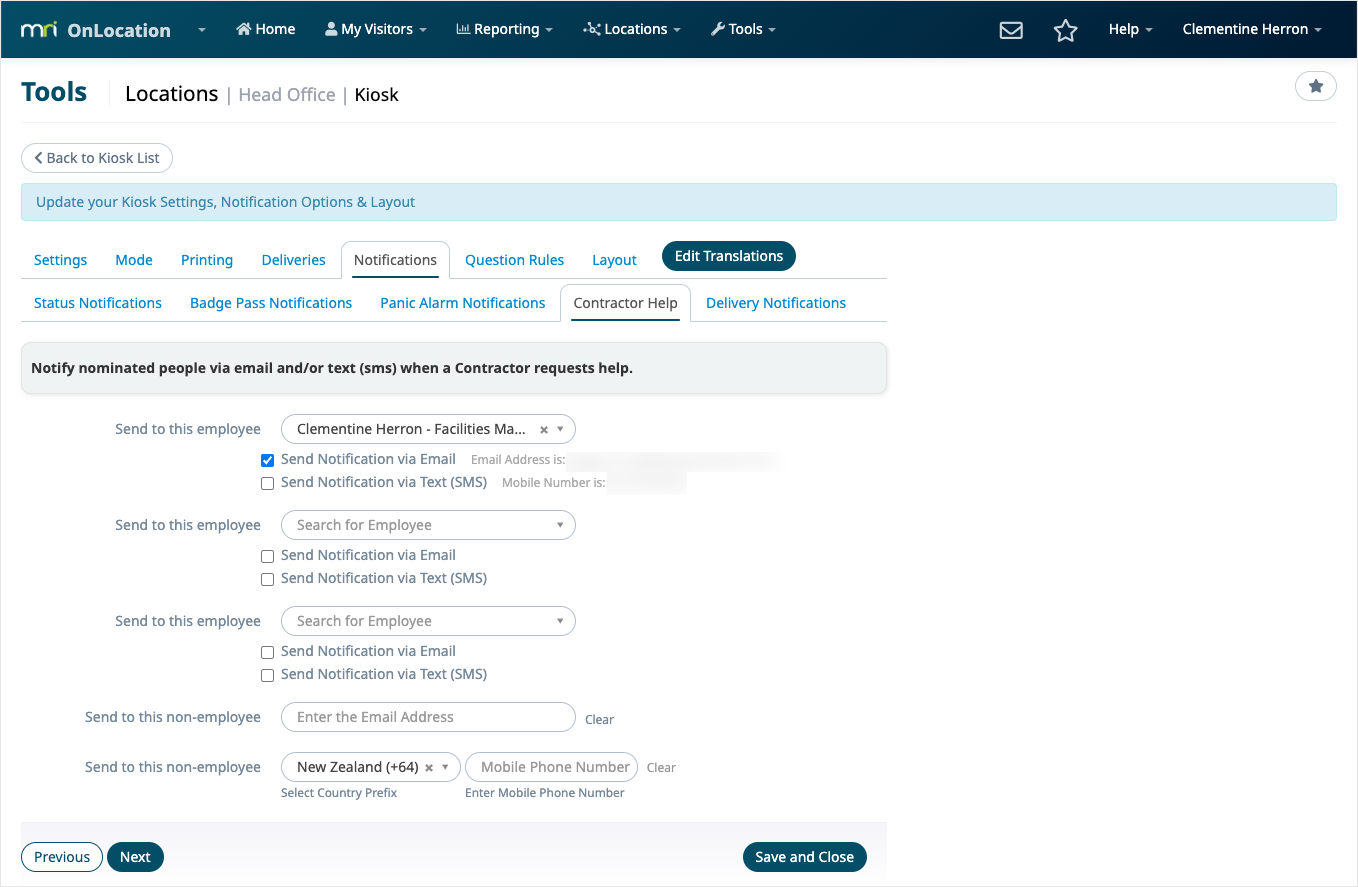This screenshot captures a detailed view of a website interface related to MRI On Location, presumably a management system for visitor and contractor notifications. At the top of the image, a dark-colored banner displays white text with navigation options such as "Home," "My Visitors," "Reporting," "Locations," and "Tools." Alongside these, there are icons for email, a star (possibly a favorites marker), help, and the user name "Clementine Herron."

Below the navigation bar, the word "Tools" is prominently displayed, followed by links to "Locations," "Head Office," and "Kiosk." A noticeable oblong button labeled "Back to Kiosk List" with a left-pointing arrow can be seen. Several other options are listed for managing kiosk settings, including "Update Your Kiosk Settings," "Notification Options," and "Layout."

Currently, the "Notifications" tab is selected, presenting a list of specific notification settings such as "Question Rules," "Layout," "Edit Translations," "Status Notifications," "Badge Pass Notifications," "Panic Alarm Notifications," "Contractor Help," and "Delivery Notifications." There is an emphasis on notifying nominated people via email and/or text (SMS) when a contractor requests assistance.

The page indicates that notifications will be sent to Clementine Herron, the Facilities Manager. Both options for sending notifications via email and text are available, with the email checkbox being checked. Personal contact information fields for email and mobile number are present but blurred out for privacy.

Further down, there are additional fields for sending notifications either to other employees or non-employees. For employees, options include searching for the employee and selecting notification methods (email or text). For non-employees, the user can enter an email address or select a country prefix followed by a mobile phone number. 

At the bottom left corner, navigation buttons "Previous" and "Next" are visible, and at the bottom right corner is the "Save and Close" button for submitting the changes made on the page.